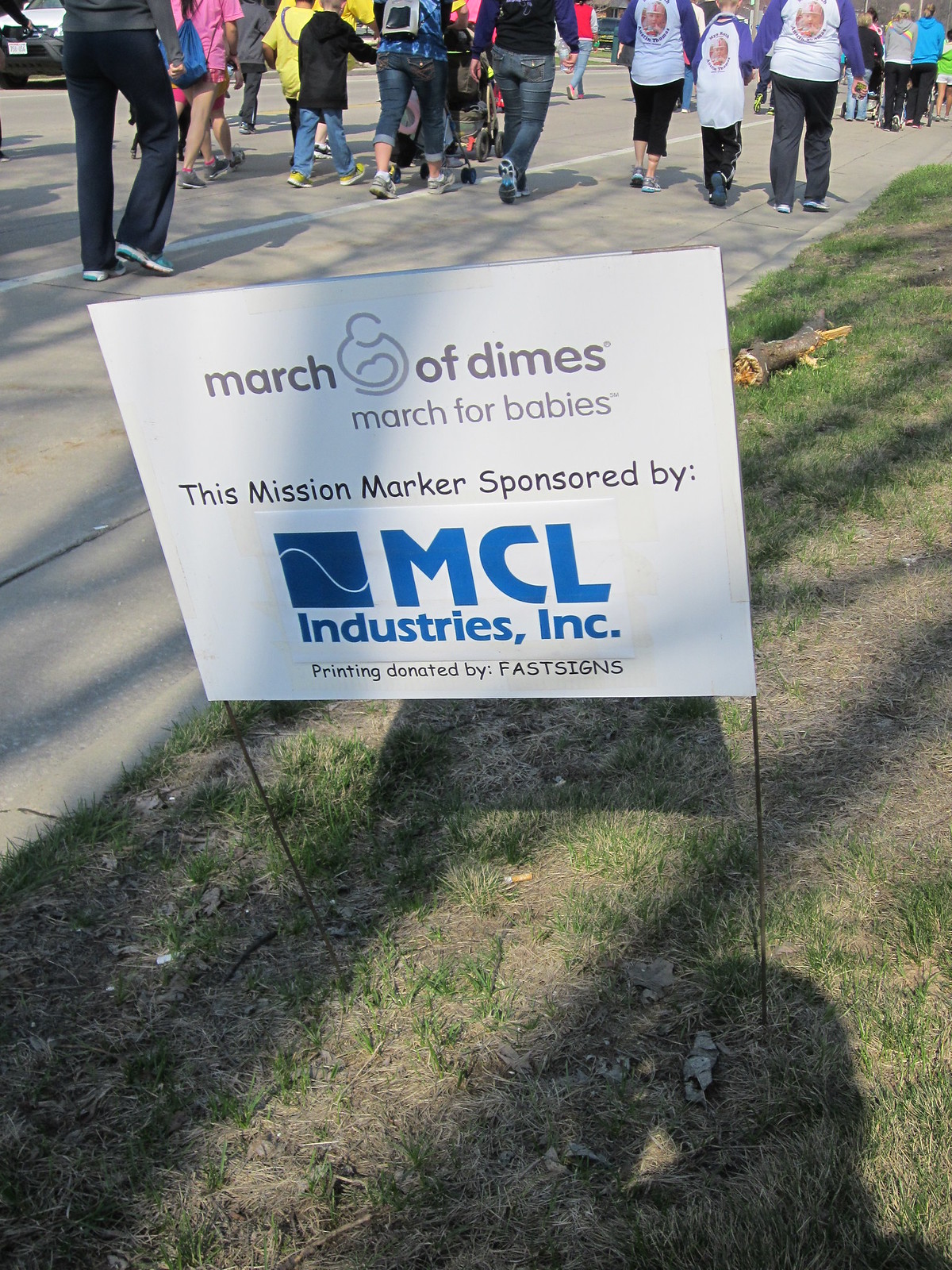The photograph captures an outdoor scene centered around a sign embedded in a grassy area near a road. The sign prominently displays the message "March of Dimes, March for Babies," with a logo that includes a woman holding a baby between the words "March" and "of." The text details that the mission marker is sponsored by MCL Industries Inc., with printing services donated by Fast Signs. Most of the sign's text is in black, while the MCL Industries portion is highlighted in bold blue, accompanied by a blue trend line as part of the logo. The scene is bustling with activity; a large crowd of people, including families with children and individuals pushing strollers, walks away from the camera along the road. The majority of people are dressed in t-shirts and either jeans or black pants, with some donning brightly colored attire. The individuals’ backs and lower bodies are visible, further emphasizing the sign as the focal point of the image. The gathering appears to be part of a parade or organized march, reinforcing the community-driven spirit of the event.